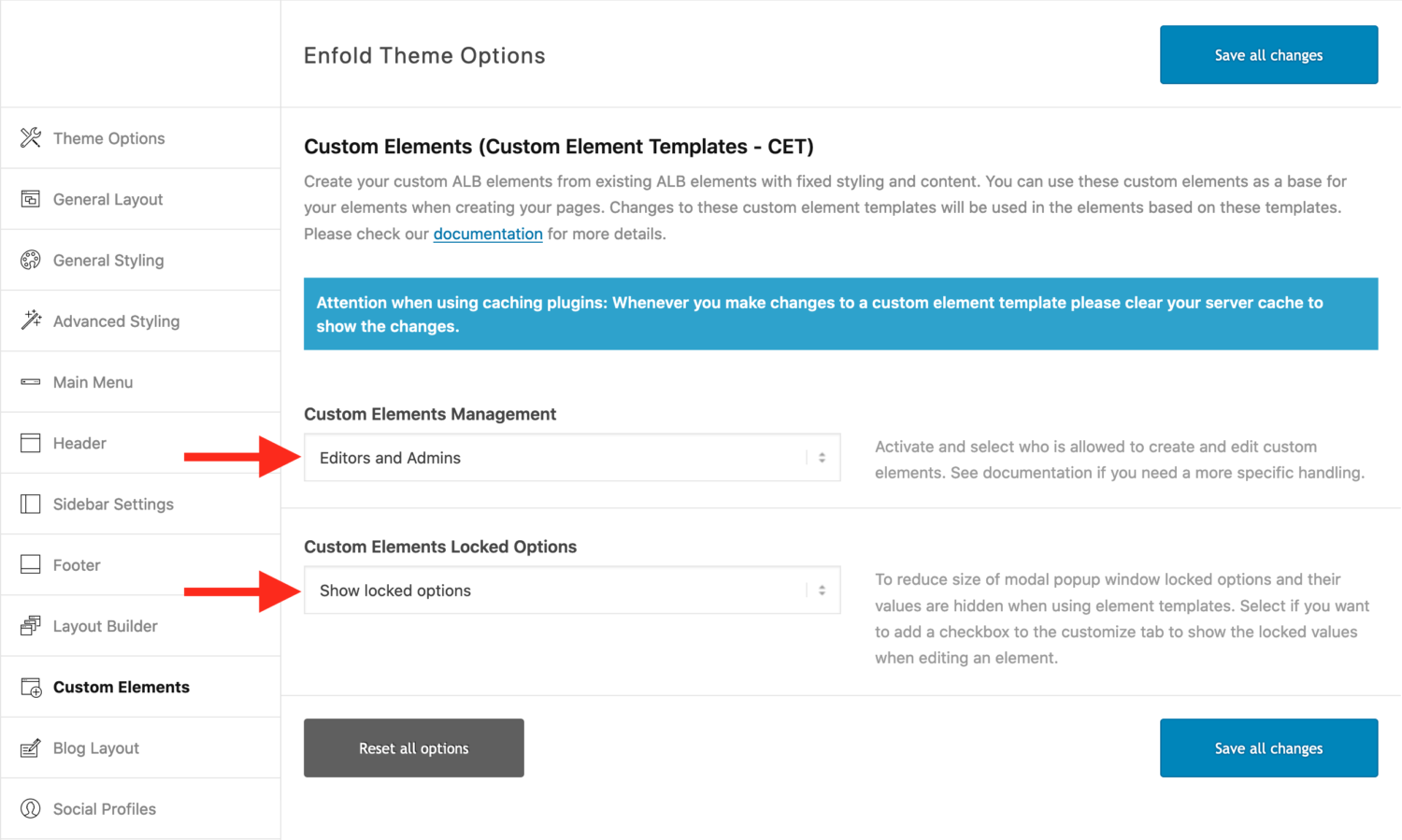This screenshot captures the administrative backend of a website, focusing on the dashboard interface. In the top-left corner, the label "Theme Options" is clearly visible. To the right of it, there is a prominent rectangular blue button labeled "Save All Changes."

The left sidebar features twelve distinct buttons, each accompanied by an icon on the left and corresponding text on the right. These buttons are listed as follows: Theme Options, General Layout, General Styling, Advanced Styling, Main Menu, Header, Sidebar Settings, Footer, Layout Builder, Custom Elements, Blog Layout, and Social Profiles. The buttons labeled "Footer" and "Header" are highlighted with a red arrow pointing toward the middle section of the dashboard.

In the middle section, dropdown boxes labeled "Editors" and "Admins" are visible, along with an option to "Show Locked Options." At the bottom of this section, there is a "Reset All Options" button located on the left side, and another "Save All Changes" button on the right side.